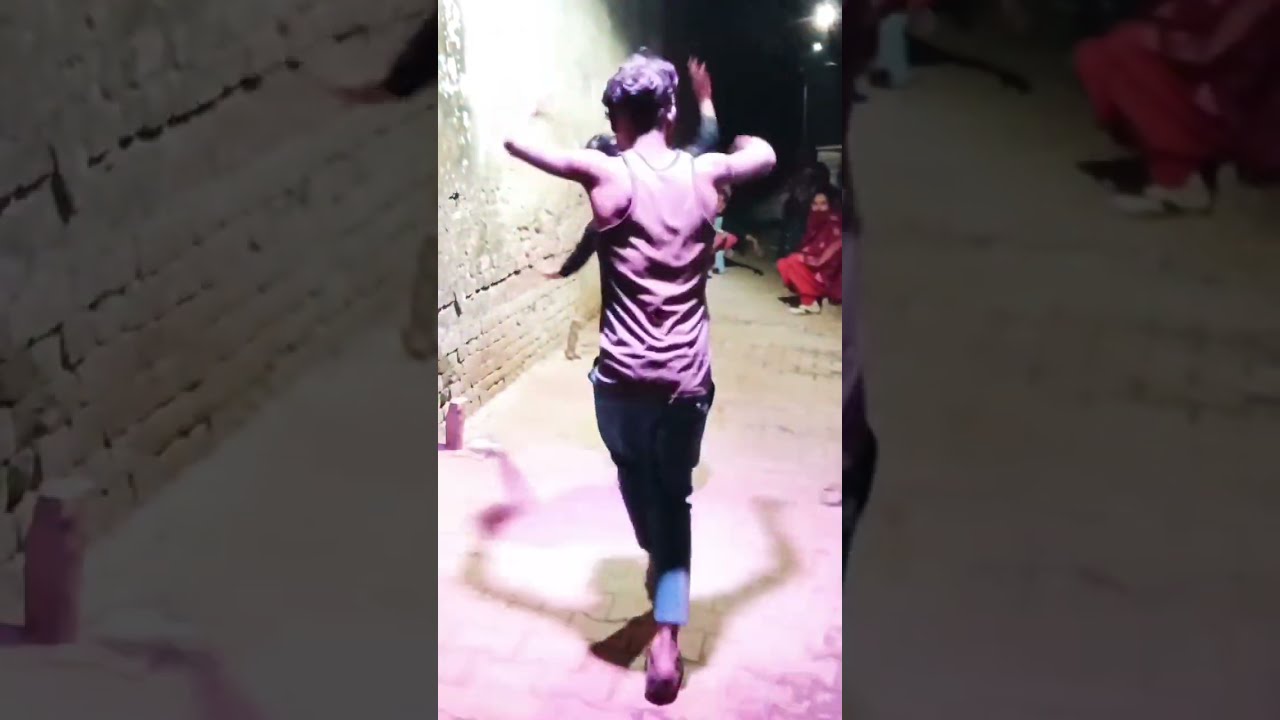In this image, we see a dynamic scene set in what appears to be an outdoor alley or street, possibly in a foreign country such as India. Central to the image is a lean, muscular man who looks like he is dancing. He has his arms extended outward, reminiscent of someone about to dive, and is notably clad in bell-bottom pants and clogs. He is walking away from the camera, positioned directly in the center of the frame.

The ground beneath him is a stone or concrete pavement, and the surrounding environment includes a discolored tan brick wall on the left, suggesting an old building. The overall scene is dimly lit by street lamps, casting a shadow that elongates and distorts the man's figure on the ground.

In the darker, almost rectangle-shaped background, which appears like a close-up from a mobile app screenshot, a woman kneels in the back right corner of the main image. She is wearing a red gown with different colored red pants and white shoes, looking towards the central dancer. Behind him, another dancer is partially visible; only his head with a bald spot, some black hair, and his raised arms can be seen. Additional figures are kneeling or sitting on the ground at the distant end of the alley, completing this nocturnal, vibrant scene captured in hues of tan, gray, white, purple, pink, red, and black.